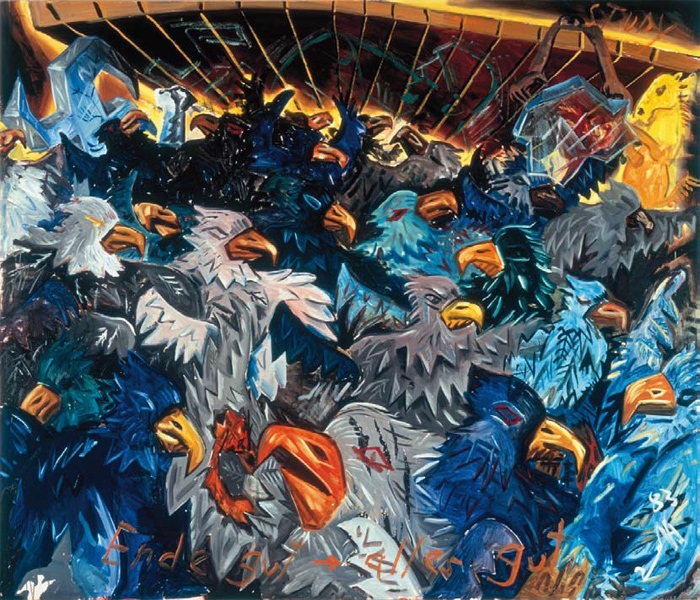The detailed illustration depicts a chaotic and visually dense scene of numerous birds, primarily resembling eagles and vultures, in a myriad of colors including blue, black, white, gray, and indigo, with their vibrant golden and yellow beaks standing out against the darker hues. The birds are tightly packed together, facing various directions with intense, serious expressions. Among them, a bird in the center has a prominent red mark around its eye, while another bird to its left features a glowing yellow eye.

The backdrop of this avian frenzy is a rustic wooden platform with vertical beams overhead. To the top left, a pair of hands gripping a pointed object emerges from the background, while to the top right, a horse-like figure stands, seemingly clutching a crystalline object that shimmers blue and red. Above the birds, a hooked crystal-like structure casts an enigmatic presence.

At the apex of the image, a golden-hued cage appears, with bars so narrow they seem almost delicate, from which the birds seem to be escaping, flying out in a wave-like pattern. Near this golden cage, a small, vaguely-defined gold object—reminiscent of a mouse or statuette—adds to the intricate tableau.

Overall, the illustration exudes a sense of entrapment and chaotic liberation, with the mass of birds embodying a mixture of desolation and urgency as they emerge from confinement.